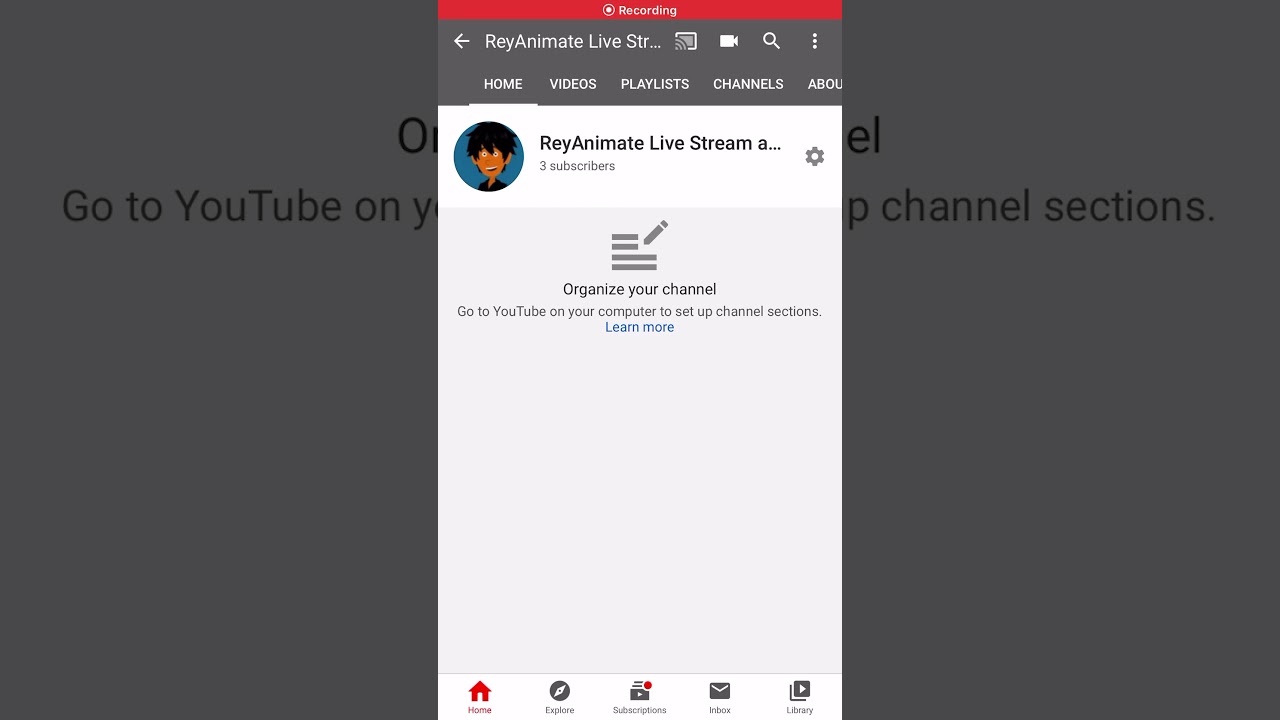This image depicts a webpage with a dark overlay that obscures the text. Despite the overlay, some of the black text remains partially legible, reading "Go to YouTube On," followed by another obscured section, and then "Channel Sections" at the far end. Superimposed on the main image, there is a screenshot of a cell phone screen marked by a red border at the top that says "Recording." Below the border, there is a left-pointing arrow next to the words "RayAnimateLiveSTR...". The interface includes icons for a video camera, a magnifying glass, and a menu with three vertical dots. The navigation options "Home," "Videos," "Playlists," "Channels," and a truncated "About" follow, with "Home" being the selected and underlined option.

In the white background area below, there is a circular avatar on the left showing an animated picture of a man's face with the label "RayAnimateLiveStreamA..." next to it. Beneath this, the text "Three Subscribers" appears smaller in size, alongside a gear icon on the right.

Further below, against a gray background, a pencil icon is accompanied by four horizontal lines and the text, "Organize Your Channel. Go to YouTube on your computer to set up channel sections."